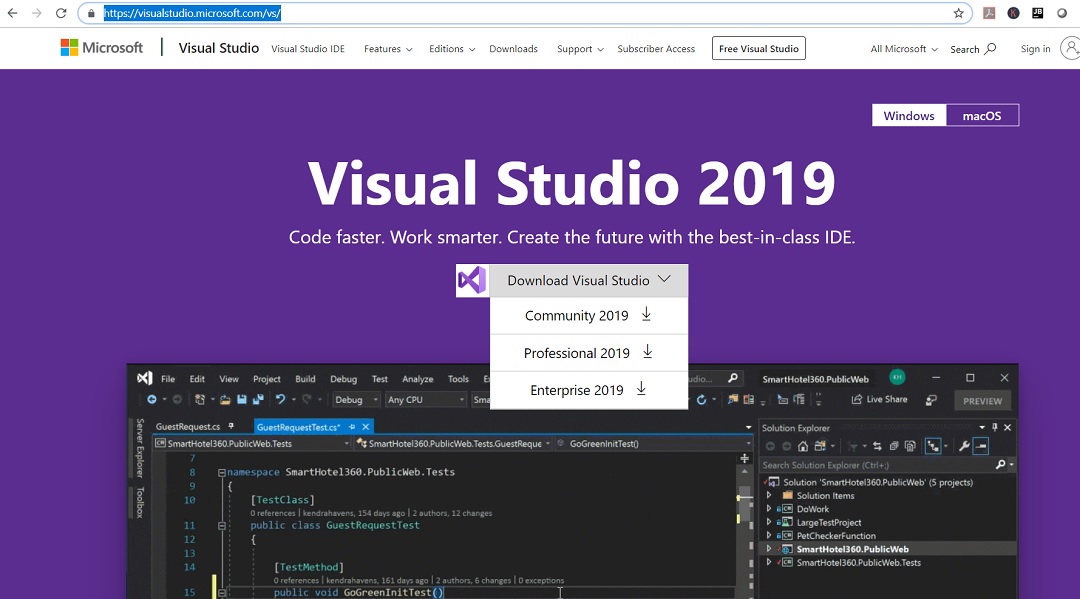**Detailed Caption:**

This is a detailed screenshot of the Microsoft Visual Studio 2019 webpage. The page boasts a sleek purple background with prominent white text, highlighting its flagship IDE with the slogan: "Visual Studio 2019, Code Faster, Work Smarter, Create the Future with the Best in Class IDE." Below the slogan is a drop-down menu offering download options for three different editions: Visual Studio Community 2019, Professional 2019, and Enterprise 2019. In the lower half of the screenshot, there's an image of a partially displayed code editor featuring a black background filled with numerous coding elements and interface components. At the top of this section is a white menu bar. Situated on the far left, it prominently features the Microsoft logo. The menu options displayed across the bar include Visual Studio, Visual Studio IDE, Features, Editions, Downloads, Support, and Subscribe.